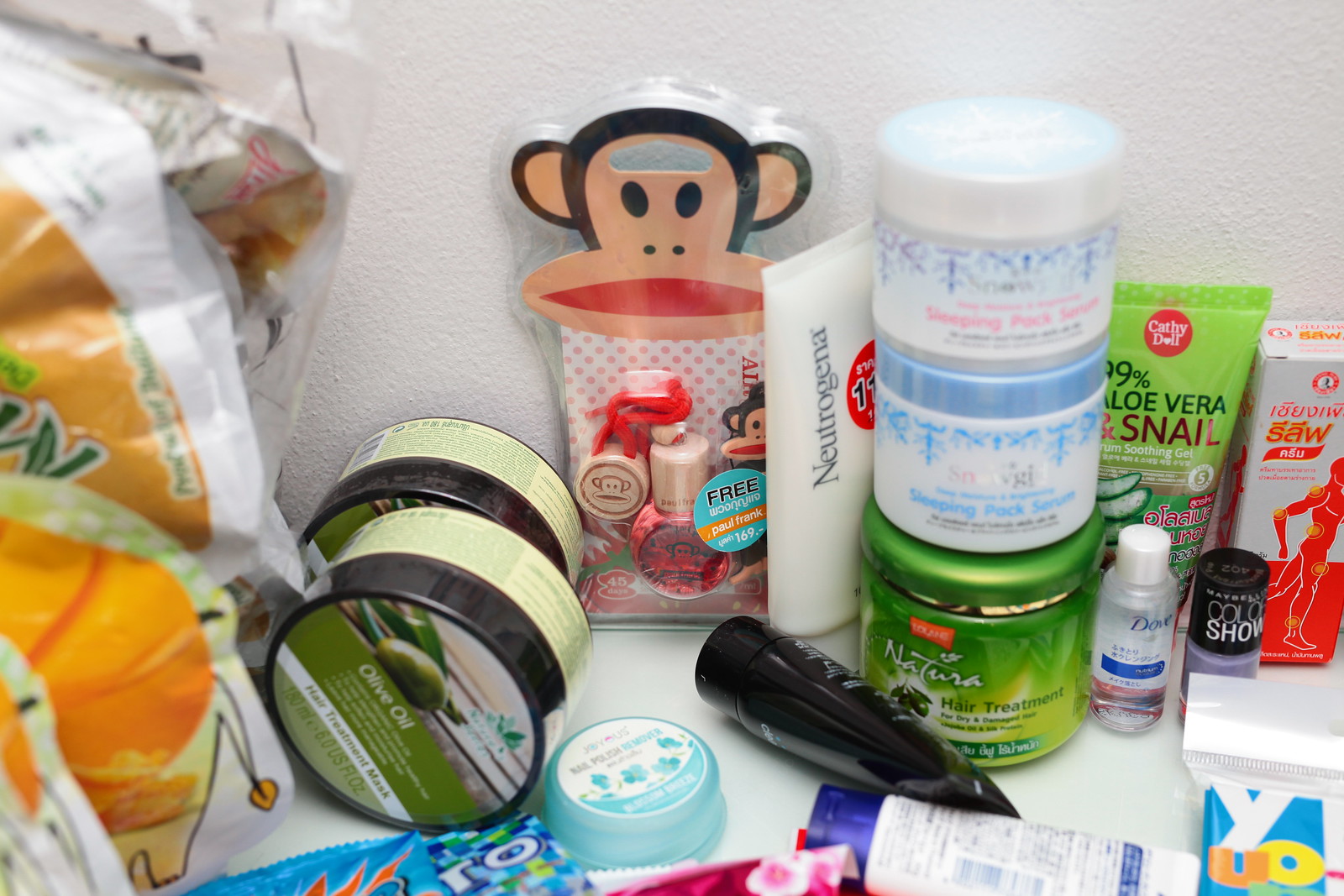The photograph depicts an organized shelf inside a white closet, filled with various health care and hygiene items. On the left side of the shelf, there are several plastic bags, each featuring an orange-colored image of what appears to be animals, including an elephant or lion. Adjacent to these bags are two round, short jars lying on their sides, labeled "Olive Oil," suggesting they contain a lotion or similar product. 

Moving right, there is a plastic container with a cartoon monkey's face on it, housing smaller items, possibly nail polishes, including a smaller matching monkey figure inside. Nearby, a short black tube rests on its side, although its label is unreadable. 

Next, a prominently displayed jar of Natura hair treatment with a green label sits beneath two stacked jars of "Snow Girl" sleeping pack serum—one with blue icicle imagery and the other with pink lettering. To the right of these, a green tube labeled "99% Aloe Vera Prescription Snail" soothing gel stands upright. 

Further right is a white and orange box with a person logo, likely from Arm & Hammer, though its non-English text leaves its content unclear. Next to it, a small bottle of Dove with clear contents is also labeled in a non-English language. Between the monkey container and the sleeping pack serums stands a tube of Neutrogena lotion upright.

The bottom portion of the image shows several other tubes and hygiene items, some partially cut off and others lying on their sides, completing the assortment of personal care products on the shelf.